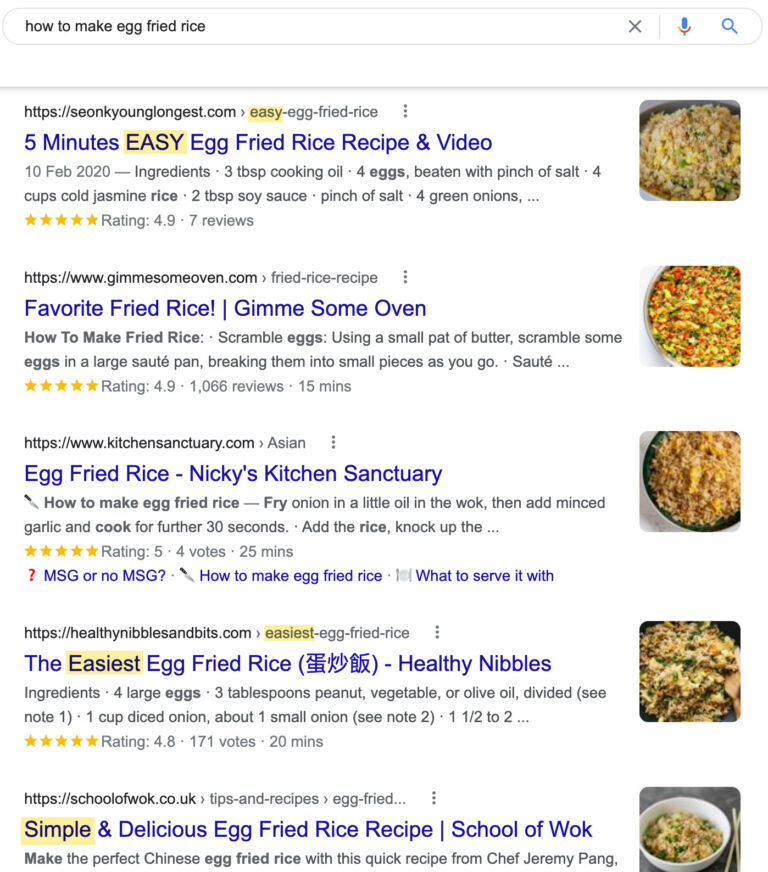The image depicts an online search for "how to make egg fried rice." At the top of the page is the search bar displaying the query. Below the search bar are five different websites listed, each offering a recipe for egg fried rice. The first result is titled "Five-Minute Easy Egg Fried Rice Recipe and Video," dated 10 February 2020. It includes a quick list of ingredients: three tablespoons of cooking oil, four eggs beaten with a pinch of salt, four cups of cold jasmine rice, two tablespoons of soy sauce, a pinch of salt, and four green onions. 

The second result is "Favorite Fried Rice" from the website "Gimme Some Oven." The third link is "Egg Fried Rice" from "Nikki's Kitchen Sanctuary." The fourth result is titled "The Easiest Egg Fried Rice" from a source with Asian writing and noted as "Healthy Nibbles." The fifth and final result is "Simple and Delicious Egg Fried Rice Recipe" from "School of Wok."

On the right side of each search result is a box containing an image of egg fried rice presented in various containers and styles, composed of diverse colors and garnishes.